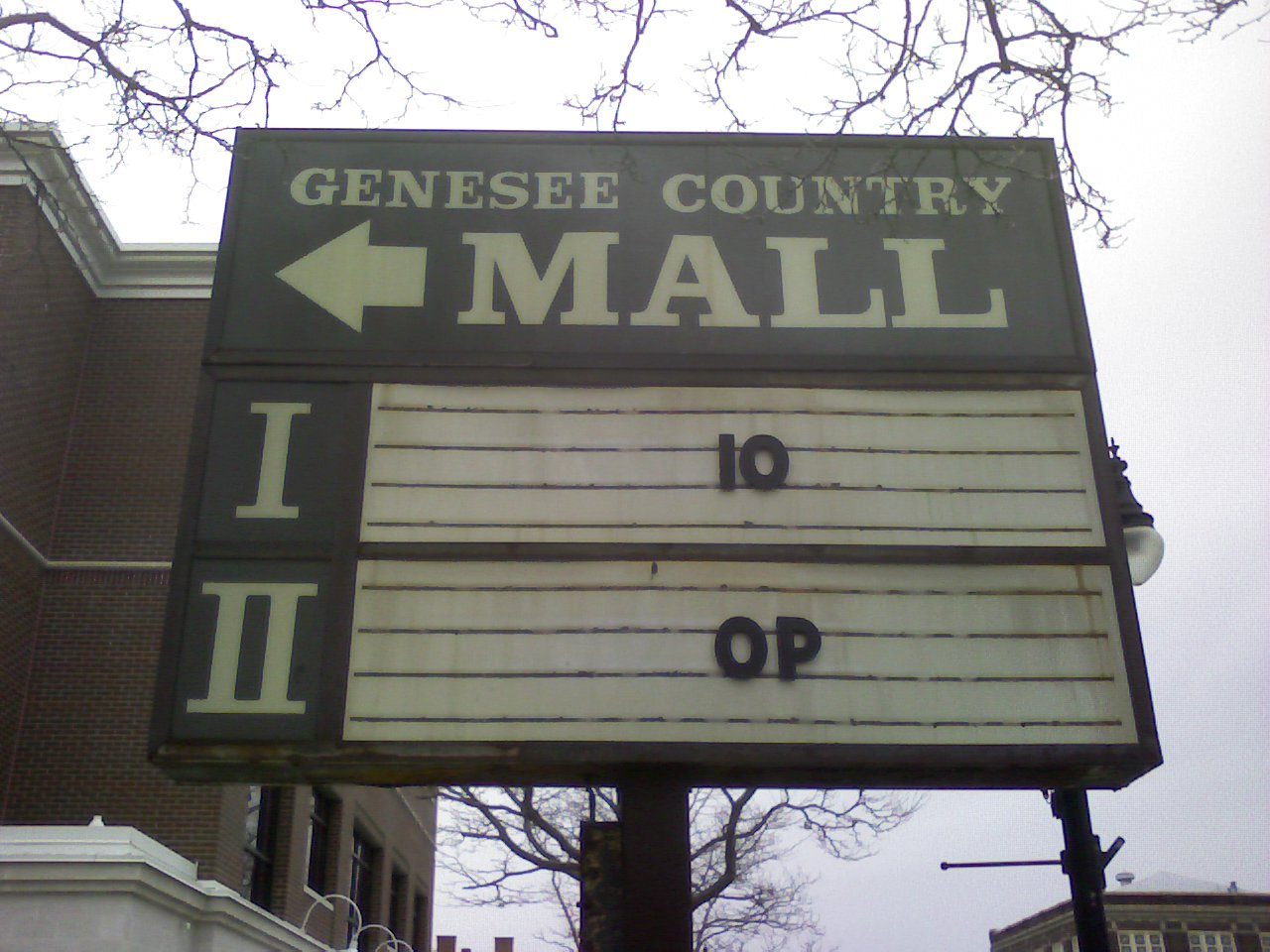The image depicts a billboard sign situated at the entrance to what appears to be an industrial park housing various businesses. The photograph is taken from a low angle, giving a slightly upward and slanted perspective on the sign. The sign prominently features the text "Genesee Country" in a smaller font above the word "Mall," which is displayed in a much larger font to make it more noticeable. Next to the "M" in "Mall," a solid white arrow points to the left of the image, indicating the direction. Below these main elements, there is another row of information: on the left side, the number "1" is displayed, and next to it on the right, there is a white section showing the number "10." Further below, the number "2" is visible with a white section to the right displaying the letters "OP."